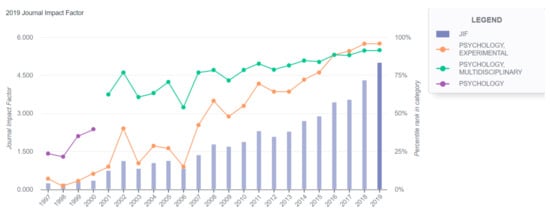The image displays a detailed combination bar and line graph illustrating data trends over time. The x-axis represents years, shown in grey bars, while the y-axis denotes an unspecified metric, with a focus on the "2019 Journal Impact Factor" as stated in the upper left corner. The y-axis text is slightly blurred but repeats this information. The legend positioned in the upper right aids in deciphering the graph, using color codes: blue squares for JIF, gold lines for Experimental Psychology, green lines for Multidisciplinary Psychology, and purple lines for general Psychology. The bars and lines increase as they progress to the right, clearly depicting the trends in journal impacts across different psychology disciplines. The graph provides thorough insight despite some text blurriness, integrating visual aids like blue, orange, and green to enhance data comprehension.